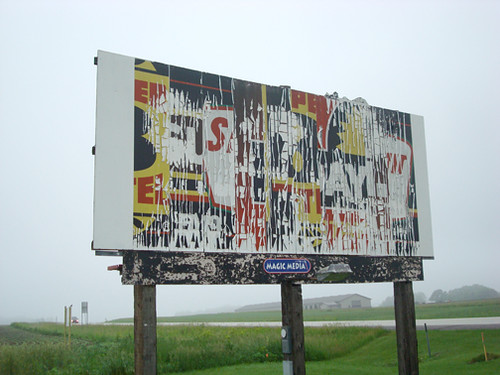This image showcases an old, weathered billboard mounted on three sturdy wooden posts. The base of the billboard is characterized by a horizontal rectangular piece of wood, which is covered in faded, chipped black paint. The faded paint attests to its age and exposure to the elements. Near the bottom of the billboard, a logo for the brand “Magic Media” is visible, proudly displaying the origins of this now outdated advertisement structure.

The main section of the billboard is no longer in active use and exhibits a complex tapestry of overlapping layers from various past advertisements. The remnants present a vibrant yet chaotic color scheme dominated by hues of orange, red, yellow, and hints of blue. Among the layered paper and paint fragments, the most distinguishable element is a faded logo that signifies a past advertisement for "Motel 8," standing out amidst the visual clutter. This scene tells the story of an era gone by, encapsulated in this solitary, decaying billboard.